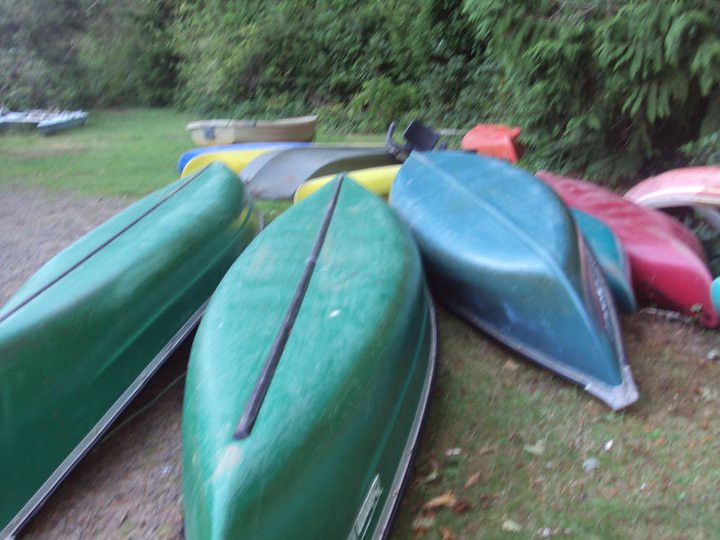The image captures a slightly blurry and desaturated scene of a collection of canoes and kayaks lying upturned on a mostly grassy area with patches of gravel, indicative of a campground or park setting, possibly near a riverbank. The foreground is dominated by two green canoes, which have a noticeable grey metal line running through their middle. Adjacent to these and further to the right is a blue canoe, followed by a red one that appears to be resting on its side. The scene is peppered with more colourful boats in the middle and background, including red, blue, and yellow kayaks, and what seems to be a small rowing boat positioned upright and beige in color. Scattered autumn leaves add to the sense of a natural, albeit somewhat unkempt, environment. In the upper left of the image, a blurred white object is faintly visible, though it's indistinct and not clearly identifiable as a boat. The backdrop is composed of either a forested area or thick hedgerow, contributing to the overall wooded, serene atmosphere of the setting.